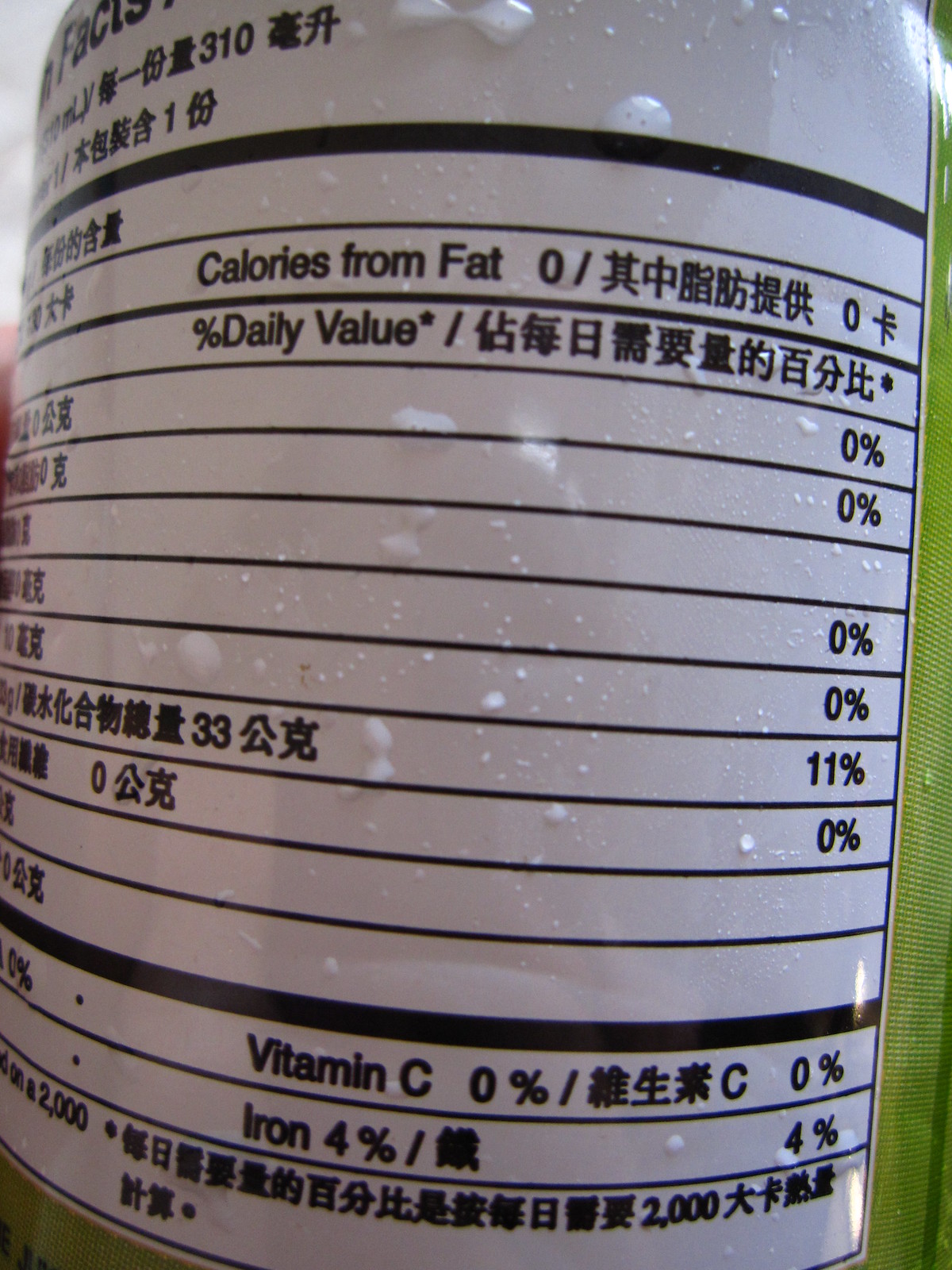A close-up view of a shiny white plastic bottle reveals its nutritional label adorned with droplets of moisture. The label, predominantly white with black lines, features a mix of Asian characters and a few English words. On the right side, a hint of green printing adds a touch of color. The label details that the product has zero calories from fat, stated in both English and Asian figures. Below, it lists the percent daily values: zero percent for most entries, including Vitamin C, with the exception of Iron, which is marked at four percent. One of the rows indicates eleven percent, standing out among the series of zeros.